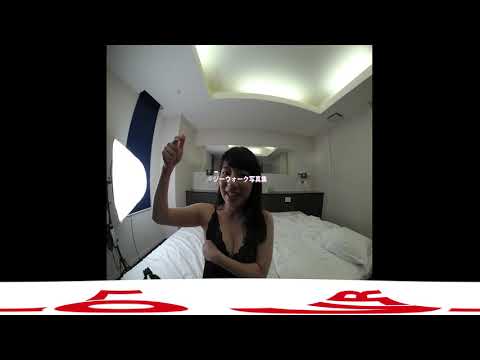The photograph features a young woman with long brown hair, parted to the side, sitting on a bed with pristine white sheets and bedding. She's taking a selfie, using one arm to possibly click a device and the other arm is crossed over her chest. The room appears to be a bedroom with white-painted walls. In the background, there is a dresser, a mirror, and some other furniture partially visible, including a long cabinet with various objects, possibly a vase with flowers. The room’s lighting comes from a lamp on her left and an architectural ceiling cutout that allows recessed light to filter through. The woman is smiling directly at the camera and is dressed in a lingerie top or negligee. The image is bordered by a heavy black frame, adorned with red angled text and an additional banner at the bottom in a foreign language. Her face is partially obscured by white text, possibly numbers or foreign writing. The overall color palette of the image includes black, white, red, dark blue, gray, and yellow. The photograph's setting is clearly indoors, capturing a private and intimate moment in her personal space.